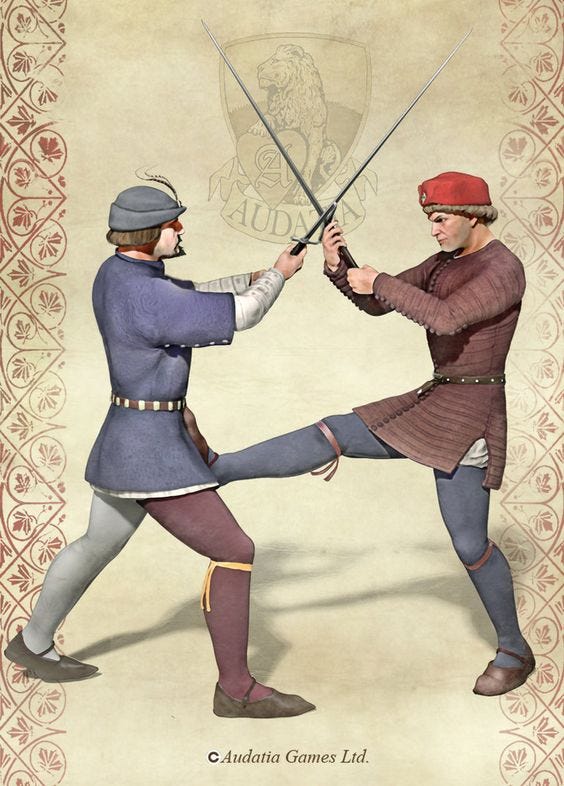This pixel art illustration by Audacia Games Limited features a medieval duel between two men, set against a light gray background with intricate ornamental scrollwork framing both sides. At the top of the image, a pale gold coat of arms with a lion's head is prominently displayed, lending a sense of regality. The central focus is on two gentlemen engaged in a sword fight, their rapiers locked in combat. The man on the left, sporting a bobbed haircut, wears an archer’s blue cap and a blue tunic cinched with a belt at the waist. He is notably outfitted in mismatched leggings—his right leg in purple adorned with a yellow ribbon just below the knee, and his left leg in gray. His opponent, positioned to the right, is dressed in a quilted purplish tunic and a stylish red hat, with both legs clad in blue stockings each tied with a ribbon just below the knee. In a dramatic pose, the man on the right has his foot pressed against the groin of his adversary, adding a dynamic element to the scene. This image, reminiscent of a book cover or perhaps a back cover, combines elements of historical fashion and action, encapsulating a vivid moment of medieval combat artistry.